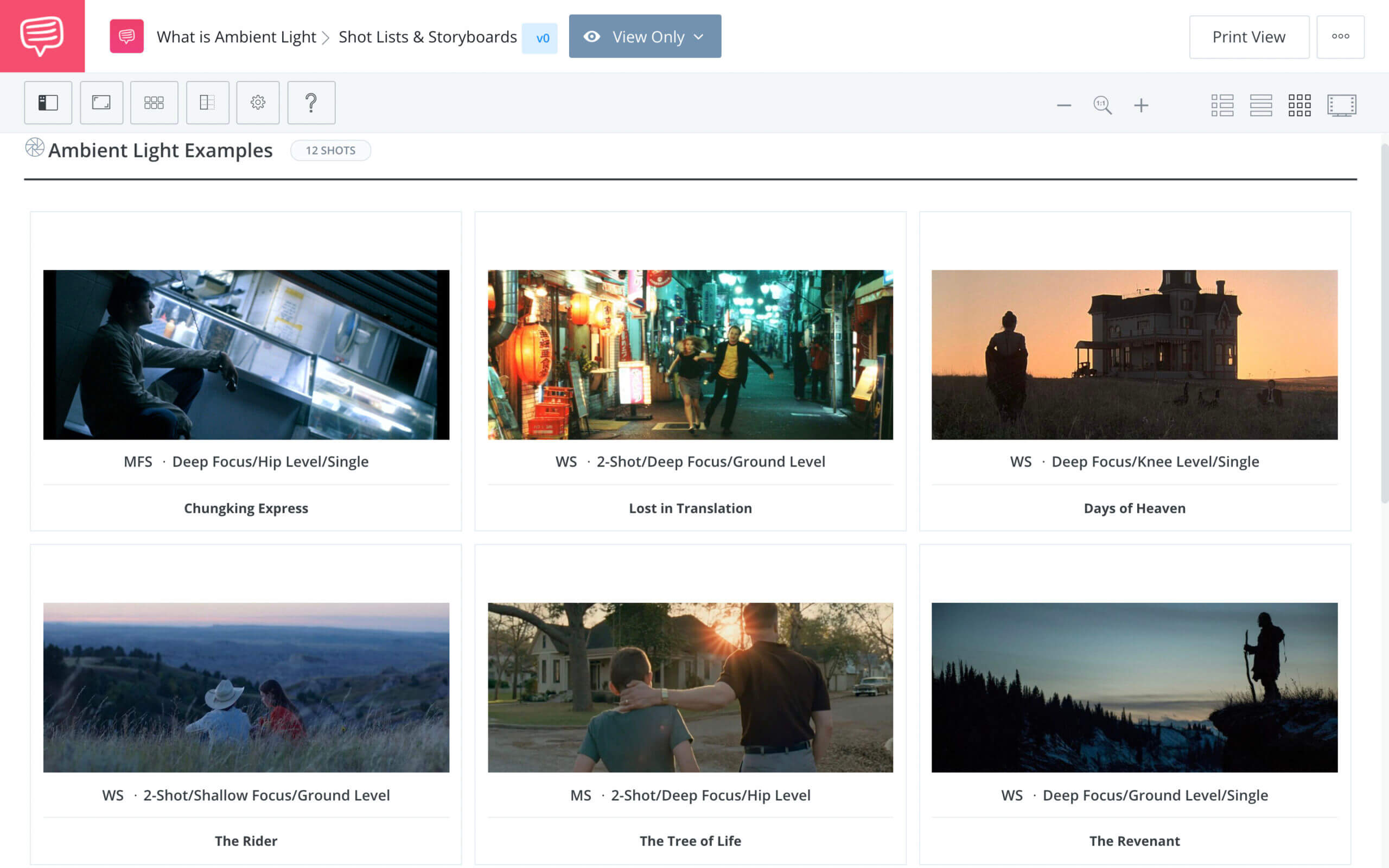The image features a predominantly white background with two pink boxes, one larger than the other, both containing white message boxes within them. To the right of these pink boxes, the phrase "What is ambient light?" is displayed in black text. Adjacent to it, a gray arrow points towards text that reads "Shot list and storyboards." Below this, there is a blue rectangle with white text stating "View Only."

On the right side of the image, there are two white rectangles — one labeled "Print Only" in black text, and the other, a square, which features the outline of three unfilled black circles, with the label "Ambient light examples" in black text. Beneath this, a gray oval containing the text "12 shots" in a darker shade of gray is present. A black line separates this section from the rest of the content.

Below the separator, there are six images with descriptive titles:

1. **"MFS deep focus / hip level single chunking express"** - Depicts a person lying against a wall.
  
2. **"WS two shots / deep focus / ground level lost in translation"** - Shows two people running in the street.
  
3. **"WSD focus / knee level / single days of heaven"** - Features a house during sunset.
  
4. **"Two shots, shallow focus, ground level, divide"** - Illustrates two people sitting surrounded by grass.
  
5. **"MS two shots / deep focus / hip level the tree of life"** - Captures two people looking at a house.
  
6. **"WSD focus / ground level / single living in it"** - Displays a person looking at grass during sunset.